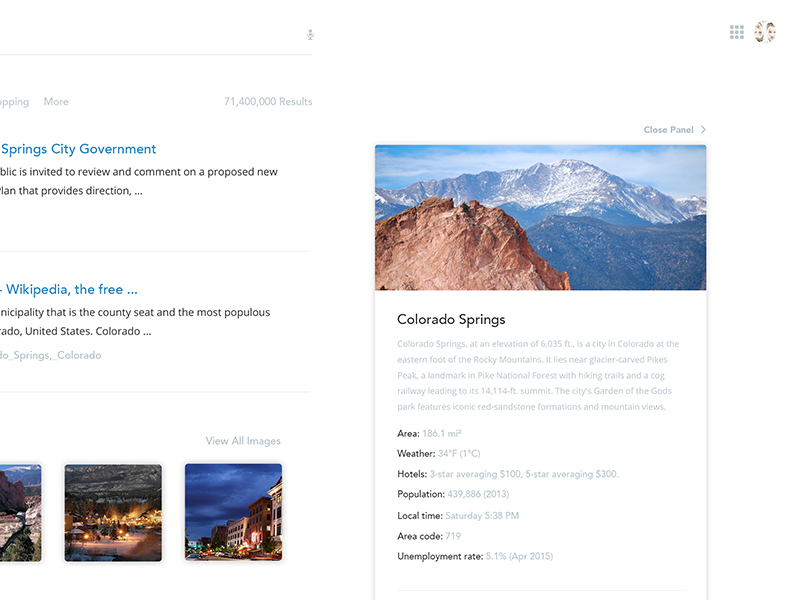The image is a vertically oriented screenshot taken from a web page, likely accessed via a smartphone or possibly a computer. The background is predominantly white, reflecting the white backdrop of the web page.

In the upper left corner, there is a gray microphone icon next to a long, thin gray line. Towards the upper right side, a dotted grid icon and a circular profile picture icon are visible. On the left, part of a cut-off word, possibly "shopping," is seen in gray text, followed by the word "more" and the number of search results, also in gray.

Below this, in blue text, the headline reads "Spring City Government," followed by additional black text providing more information. Then, in blue again, the text reads "Wikipedia, the free..." with more black text underneath providing additional details. 

A thin gray line separates sections of the content. At the bottom, there are a few images, accompanied by the gray text "View all images." 

On the right-hand side of the web page, there is a picture displaying mountains, the sky, and clouds. Above this, the words "Closed Panel" are visible. Below the image, black text reads "Colorado Springs," followed by various details about the area such as local attractions, weather, hotels, population, local time, area code, and the unemployment rate.